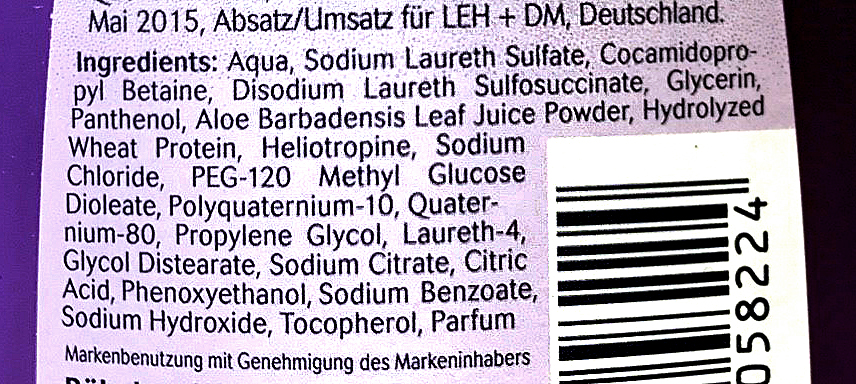This close-up image captures the back of a household item, potentially shampoo or lotion, displaying a detailed ingredients list. The background is lavender, bordered by a dark purple strip on the left and black on the right. In the bottom right corner, a white and black barcode is partially visible, with the number 058224 discernible. The list, written in black ink, includes components such as aqua, sodium laureth sulfate, cocamidopropyl betaine, disodium laureth sulfosuccinate, glycerin, and hydrolyzed wheat protein, followed by additional ingredients like polyquaternium-10 and phenoxyethanol. The text also features German words, including "Deutschland," suggesting the product may be from or intended for a German-speaking region. "MAI 2015" can be seen, likely indicating the date of manufacture or an expiration date. The presence of both English and German text indicates bilingual labeling.